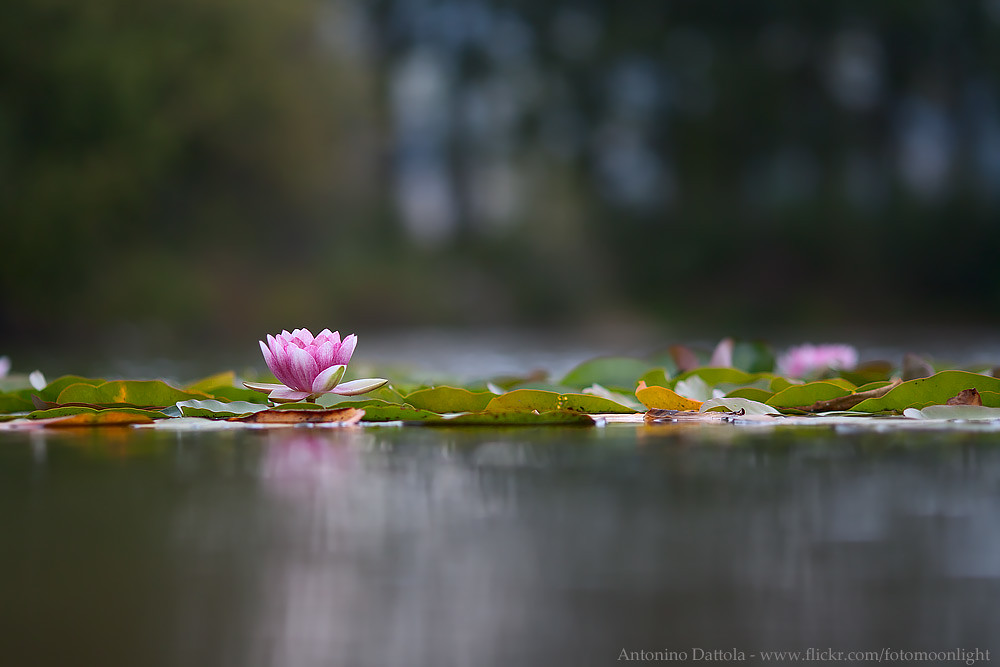This photograph, taken by Antonino Datola and available at www.flickr.com/photo/moonlight, captures an intimate and detailed portrait of a serene pond scene. The main focus of the image is a single pink and white lotus flower prominently displayed on the left side, set against a backdrop of several green lily pads. A second lotus flower, slightly out of focus, can be seen to the right, adding depth to the composition. The foreground features blurred water, suggesting the camera is positioned close to or just above the surface. In the background, although blurry, the outlines of trees and shrubs hint at a natural, tranquil setting. The photograph is marked with a watermark in the bottom right corner, crediting the photographer, Antonino Datola.